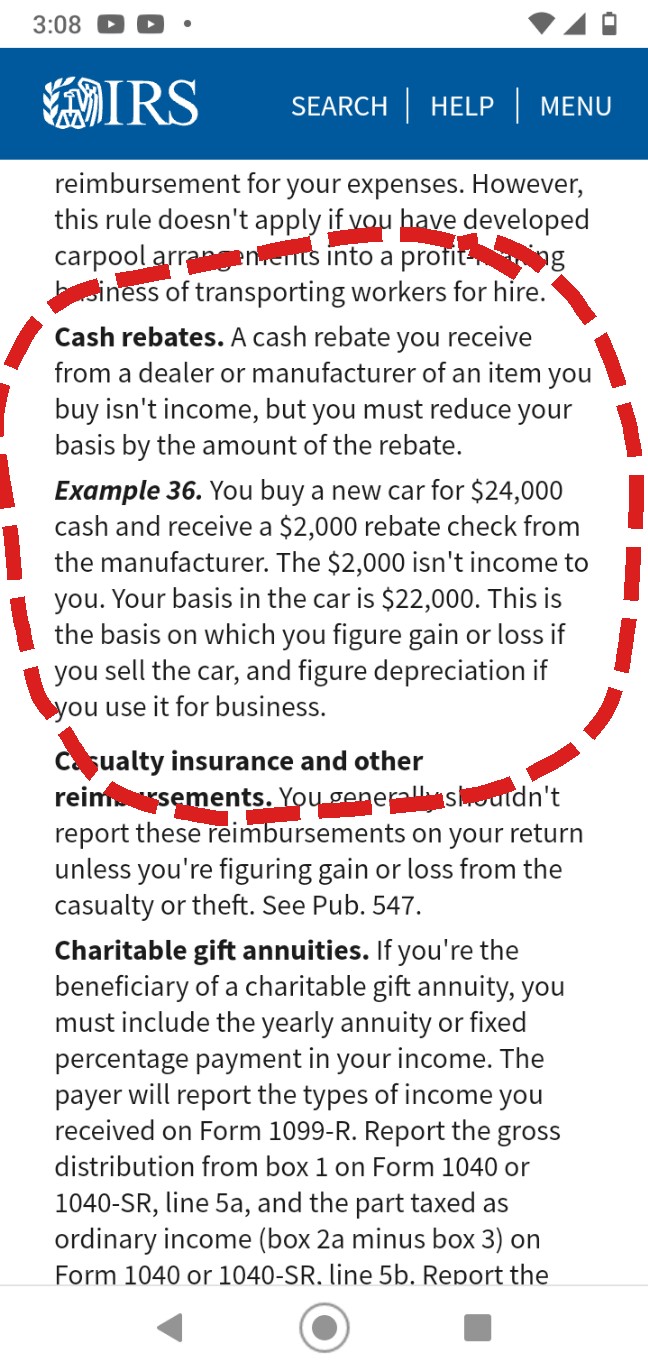A detailed screenshot of a cell phone display shows various elements on an IRS webpage. The screen proportions, about two and a half times as tall as it is wide, suggest a typical smartphone screenshot, set against a white background that obscures the exact edges of the device.

In the upper left corner, the time is displayed as 3:08 PM with two YouTube notifications beside it. The upper right corner indicates full signal strength for both wireless and Wi-Fi connections, while the battery icon displays half capacity. 

Beneath this status bar, a horizontal bar shows the IRS logo on the left with the text "IRS." To the right are navigation options: "Search," "Help," and "Menu." The screenshot captures a segment of an article, with several paragraphs of black text visible.

Key headings in bold include "Cash Rebates," "Example 36," "Casualty Insurance and Other Reimbursements," and "Charitable Gift Annuities." Notably, "Cash Rebates" and "Example 36" are encircled with a dashed dark red line, highlighting these sections amidst the text.